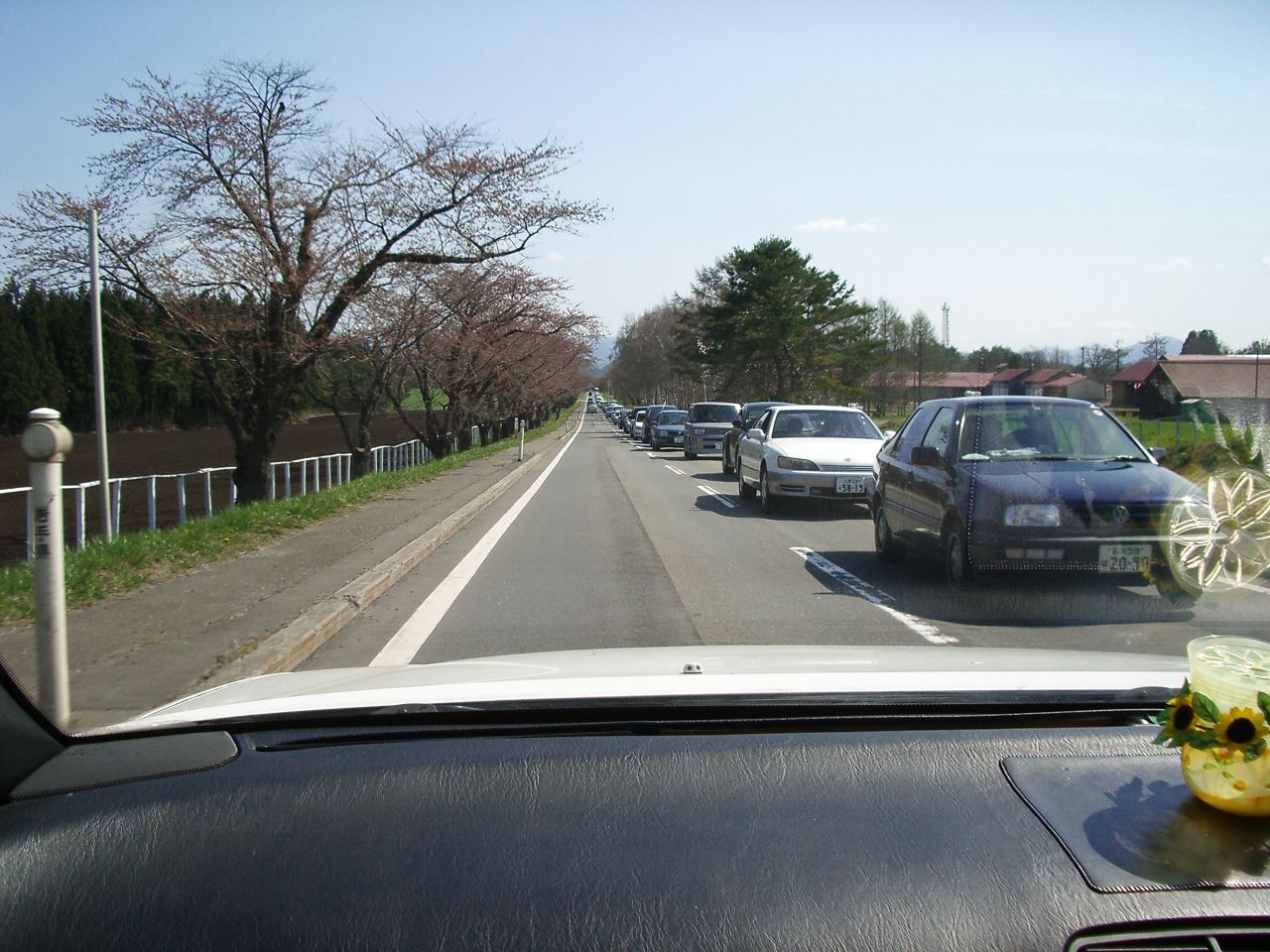A detailed photograph captures a seemingly endless procession of vehicles along a two-lane country road. The picture is taken from within a car that travels in the opposite direction, giving a clear perspective of the long line of cars queued on the other lane. The procession appears to stretch back for approximately 50 cars, eventually fading into the horizon where they become indistinguishable. 

The first car in line is black, followed by a white one, with the next few cars varying in darker colors. Among them, another white car stands out. The road is flanked by an asphalt sidewalk on the left, complemented by a stretch of grass and rows of bare trees that extend along the entire length of the road. The right side of the road features more trees, which are not as barren, with glimpses of residential homes peeking through behind them. The scene encapsulates the tranquility of a rural setting juxtaposed with the congestion of modern traffic.